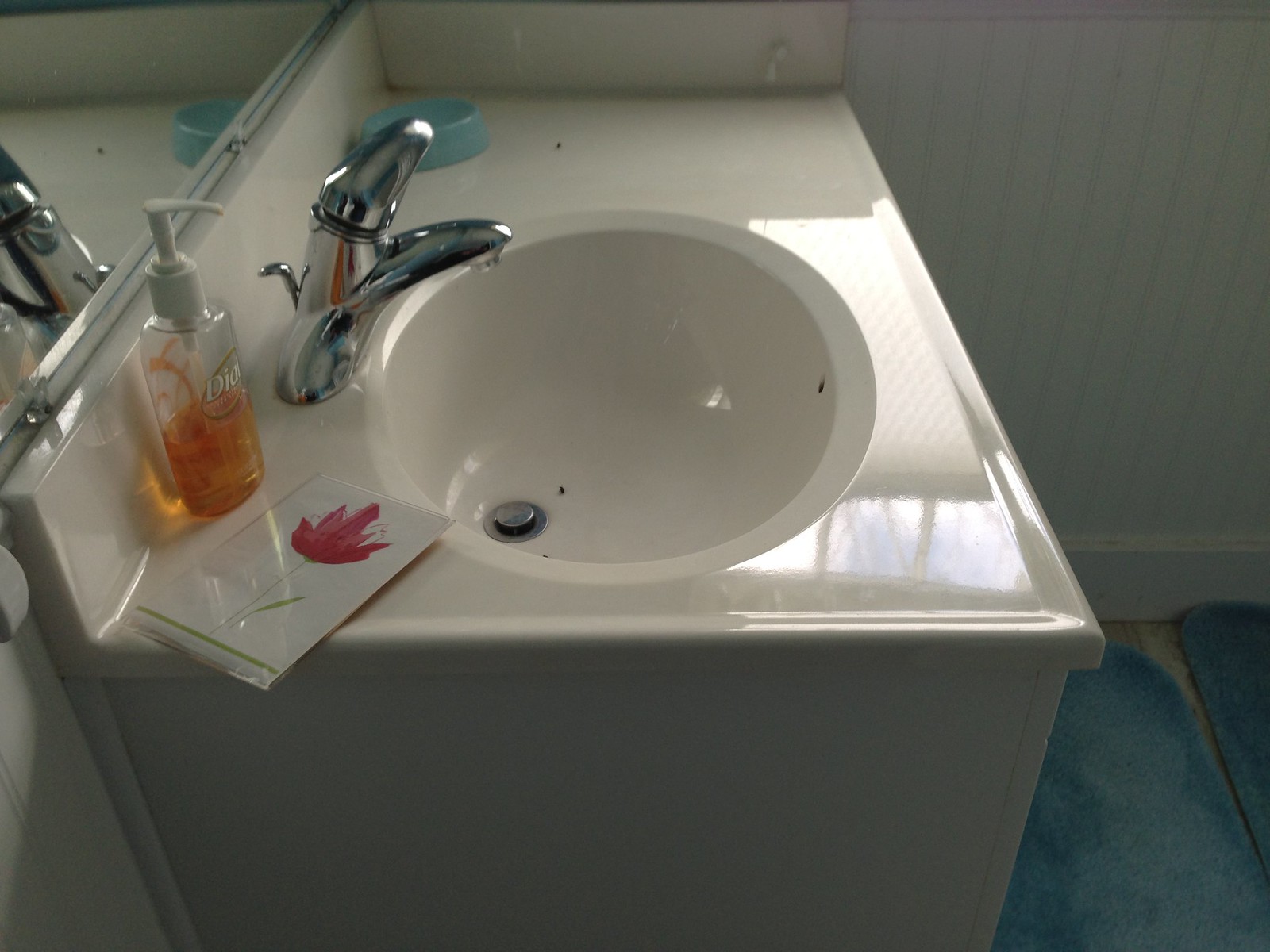This image captures a pristine white bathroom characterized by a sleek, rectangular-shaped vanity topped with a porcelain countertop. Centrally featured is a bathroom sink, viewed from the left side, showcasing its elegant design with a silver spigot and matching handle. Adjacent to the sink, on the countertop, stands a soap dispenser filled with orange liquid and bearing the "Dial" logo, topped with a white cap. 

A mirror behind the sink reflects part of the countertop and the silver spigot, adding depth to the photo. The countertop extends into a stylish six-inch porcelain backsplash that wraps around the rear and left side. On the right side of the image, a blue carpet is visible on the white-tiled floor. Additionally, the countertop houses a small blue bowl, reminiscent of one used for pet food, and a colorful card featuring a pinkish-hued flower.